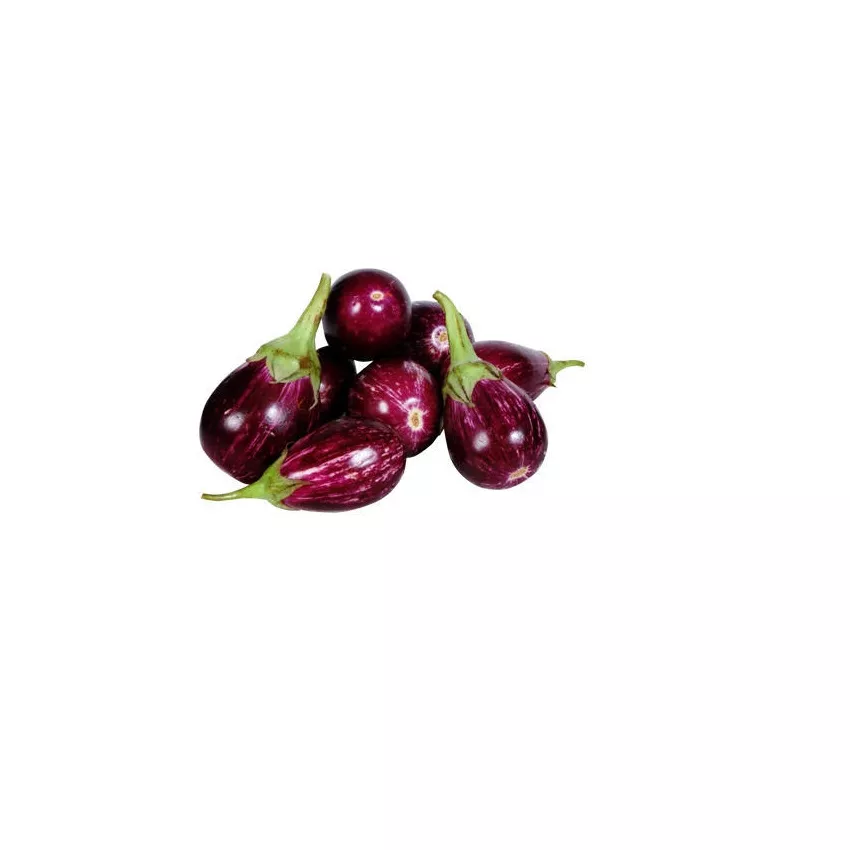The image features eight small, oval-shaped vegetables that resemble miniature or Asian eggplants. These eggplants are distinct with their lighter purple hue, accented by white streaks and spots, distinguishing them from the standard dark purple varieties commonly seen in the United States. The vegetables have a glossy sheen, suggesting they are freshly picked. Each vegetable has a green stem that looks like an upside-down tulip stem; some stems are pointing outward to the sides, especially the ones on the left and right edges, while others are directed towards the back of the image. They are arranged in a seemingly random pile, some lying flat while others are stacked on top. The background is all white, and the vegetables are illuminated by the light source within the room, enhancing their vibrant colors.